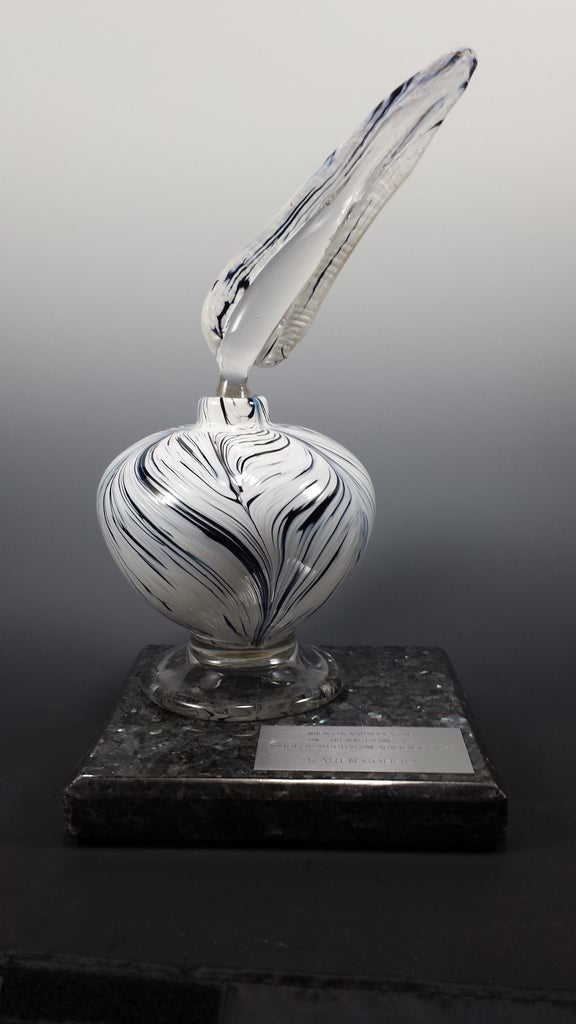The photo features a sophisticated ink and quill set positioned against a black and gray gradient background. The lower half of the image displays a sleek black slate platform, upon which rests a polished marble stand. This stand supports an exquisite, hand-blown glass vase, designed with white and blue marbled swirls, giving it an opaque, swirling effect. Emanating from the vase is a crystal-clear glass quill, crafted with intricate rivets that mimic the delicate shape of a feather, angled slightly to the left. Adjacent to the vase is a shiny silver plaque, though its inscription remains blurry and unreadable, it suggests an air of distinction, perhaps denoting an award or special recognition. The entire setup exudes an aura of elegance and luxury, reminiscent of a prized collectible or a prestigious gift.